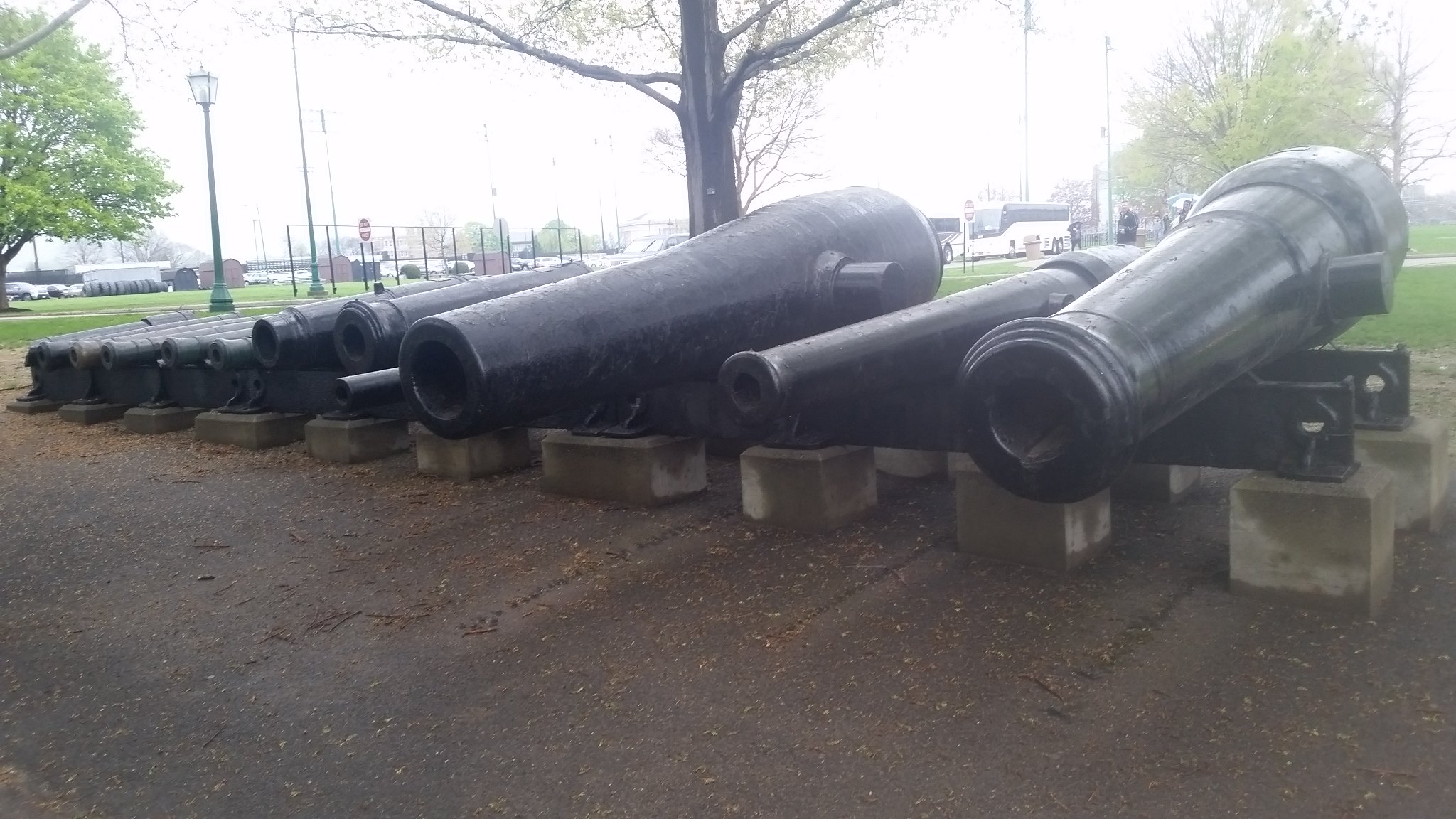This outdoor color photograph depicts a historical site, possibly a park, featuring a line of well-preserved black cannons of various sizes. The cannons are positioned on concrete bases and a dirt surface, and they descend diagonally from the right foreground towards the left. The first cannon is notably large, followed by alternating smaller and larger ones, eventually leading to five uniform, smaller cannons. The scene unfolds under a cloudy sky with white overcast, suggesting recent rain. The background shows a mix of trees with green and red foliage, some sparse enough to reveal branches. Beyond the trees, white coach buses with gray or black trim and fencing can be seen. There's also green grass and several people walking around, enhancing the lively, yet historical ambiance of the park.